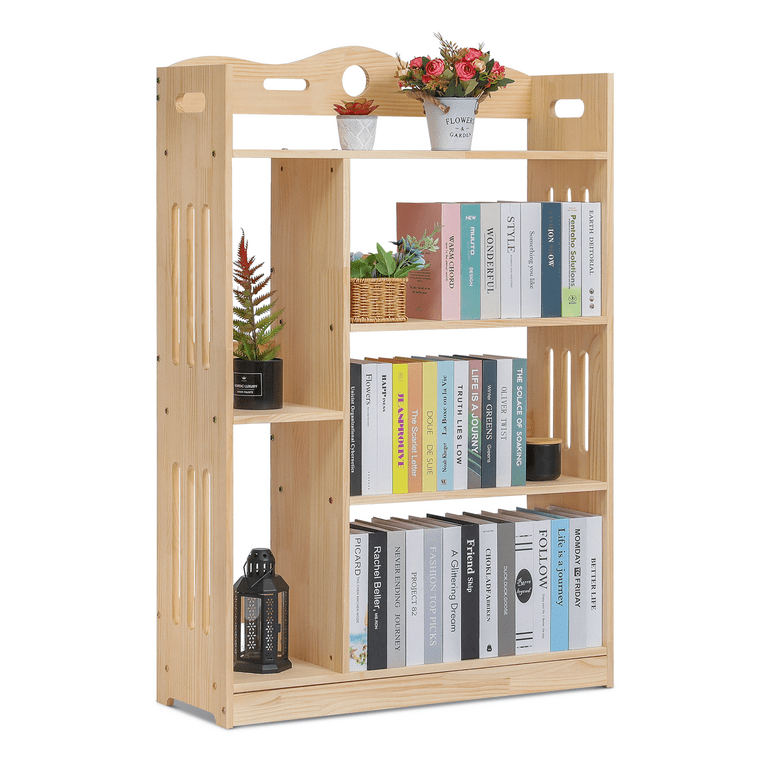A wooden shelf unit, showcasing its sturdy construction with visible nuts and bolts, stands against a light background. The wood is a light, natural tone, adding a touch of minimalism and elegance to the decor. At the very top, two charming flower pots adorn the highest shelf. The first pot, slightly larger, features an arrangement of artificial roses accentuated with delicate greenery and hints of baby's breath. The second, smaller pot contains a faux succulent, adding a modern touch to the rustic setting.

The second shelf holds a collection of books, their spines creating a varied tapestry of colors and textures. Nestled among the books is a brown wicker basket, which is spilling over with more greenery, bringing a fresh, natural element to the ensemble. 

Descending to the third shelf, there is yet another assortment of books. Alongside these, a sleek black dish with a wooden lid sits, likely containing a candle that promises to infuse the space with a warm, fragrant ambiance when lit.

The bottom shelf continues the theme of literary charm with more books. A small lantern, ready to cast a cozy glow, sits inside a little cubby, inviting a sense of warmth and comfort. Finally, just above this section is a small additional shelf, which hosts a lively green plant, completing the arrangement with a final touch of nature.